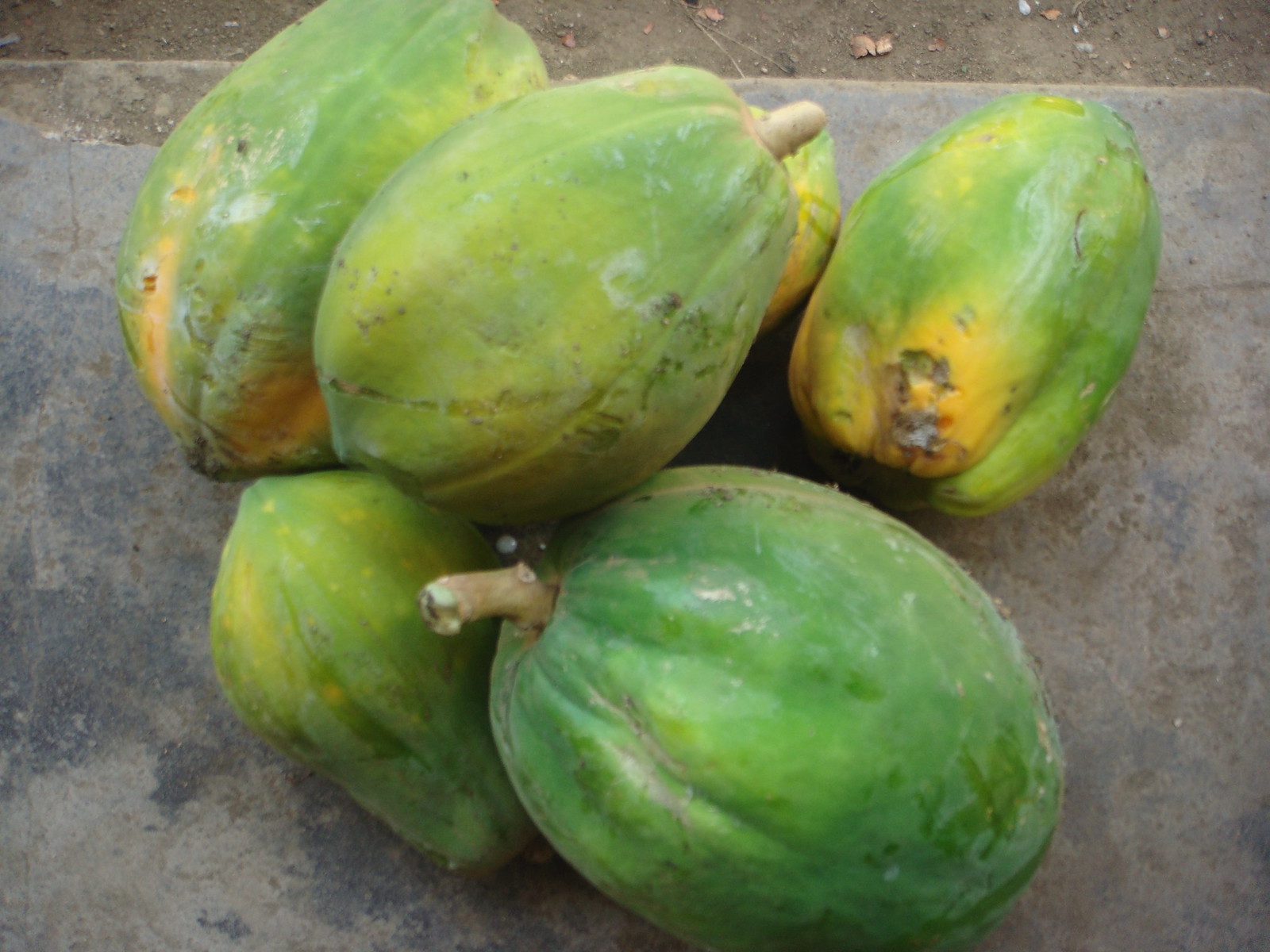In this image, we see a collection of large, green fruits, potentially melons, arranged haphazardly on a concrete step in an outdoor setting. The fruits, numbering six in total, have a predominantly bright green color, with several exhibiting gradations of yellow, especially towards the bottom. The one located on the lower right is uniformly green with patches of light green and gray spots. Others display varying degrees of yellow; for instance, the fruit in the lower left is speckled with yellow, the one in the upper left has distinct yellow spots, and the upper right fruit features a significant yellow patch with a gray circle. The fruit at the top center has a slight yellow-green tint at its bottom. Round at the base and tapering towards the top, resembling a pear shape, these fruits have brown stems. The step they rest on is a mix of black and gray cement. In the background, dirt and a few small, dried leaves are visible, reinforcing that the photograph was taken outside.